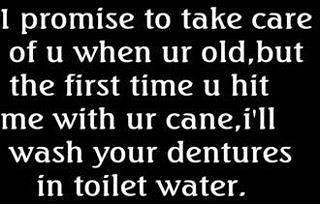The image features a striking black background with no additional elements, creating a stark contrast to the pure white text that dominates the scene. The medium-sized font is clearly legible, and displays the following playful yet amusing quote: "I promise to take care of you when you're old, but the first time you hit me with your cane, I'll wash your dentures in toilet water." The text spans multiple lines, ensuring it occupies the entire space, and is written in a straightforward, unembellished style that adds to the humorous tone of the message.